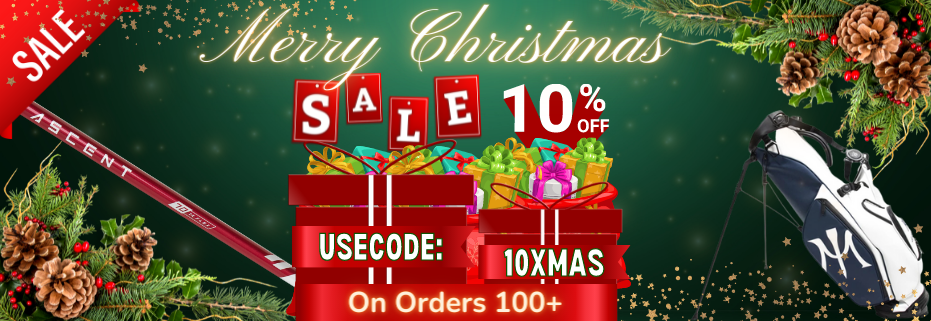This vibrant Christmas-themed advertisement showcases a festive seasonal sale. The prominent "Merry Christmas" message in bright yellow and gold stands out against a backdrop adorned with chestnut brown hues, snowy accents, pine cones, and holly leaves. Sprigs of pine needles and red holly berries add to the holiday spirit. To the left, a diagonal banner reads "Sale" in bold white letters on a red ribbon, drawing attention to the discount.

Central to the advertisement is a stylish display featuring a golf club on a navy and white stand, indicating a promotion on golf equipment. Below the "Merry Christmas" greeting, the word "SALE" is creatively displayed in a staggered manner across individual red flyers, with alternating letter heights for a playful effect.

Further down, the promotional details instruct customers to use the code "10XMAS" on purchases over $100 to avail of the special offer. This code is displayed within a decorative red present, surrounded by an array of multicolored gifts spilling out, symbolizing abundance and the excitement of the holiday season.